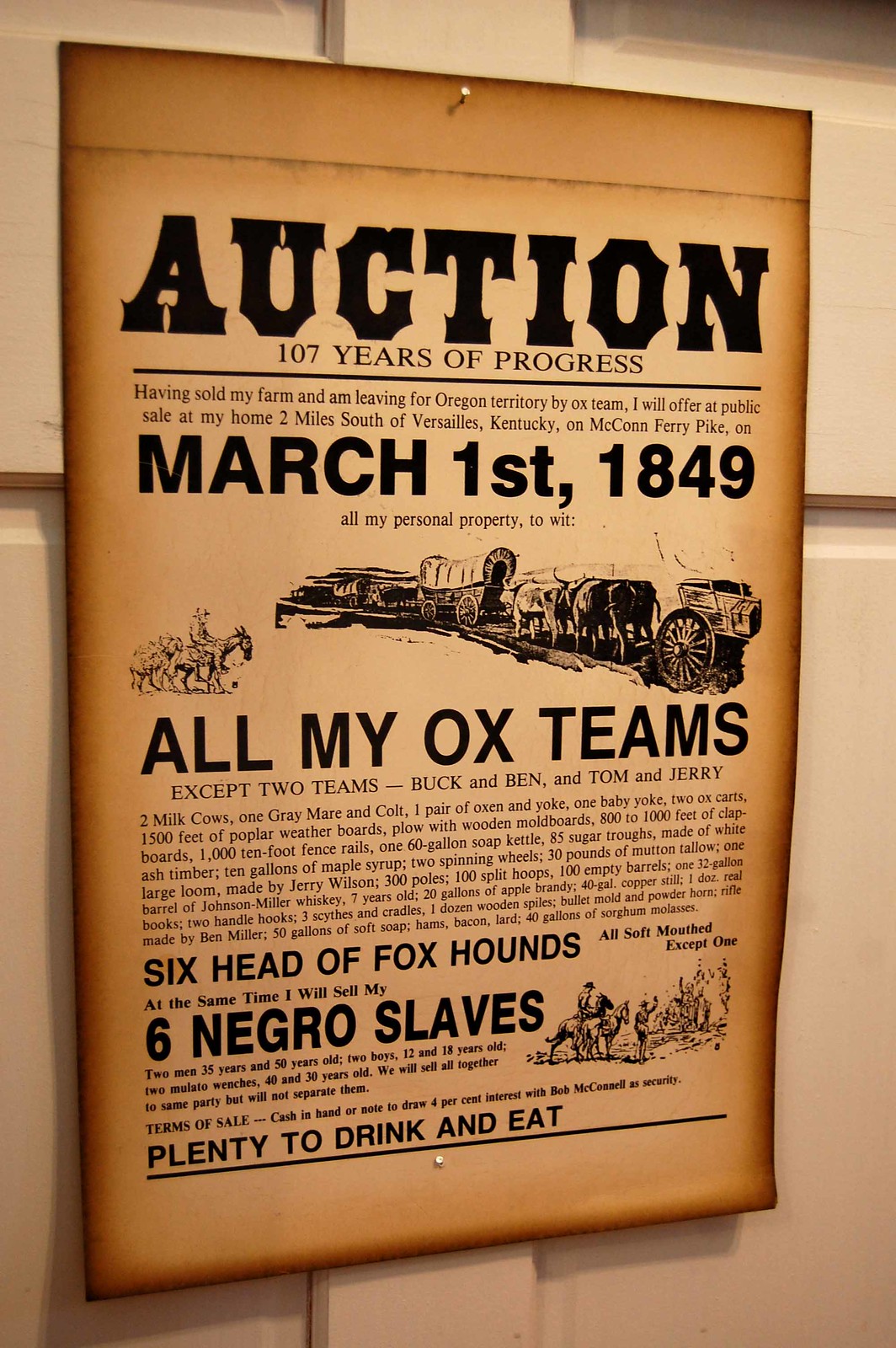This image depicts a vintage, rectangular auction poster with a worn, yellowing paper background and black text, bordered by brown and golden hues. The poster, mounted on a creamish-pinkish indoor wall, is held in place by visible nails at the top and bottom. The text, presented in various font sizes and styles, gives it an old, Wild West aesthetic complete with burnt-marked edges.

The prominent heading reads "Auction" in the largest font, followed by the subheading "107 Years of Progress," both of which are underlined. The poster announces the sale due to the owner's relocation to the Oregon Territory by ox team. The main body of the text details the auction, to be held on March 1st, 1849, at the owner's home two miles south of Versailles, Kentucky, on McConn Ferry Pike. Listed items include numerous personal properties: several ox teams except two pairs named Buck and Ben, and Tom and Jerry, two milk cows, a gray mare and colt, various farming tools, household items, and a large number of goods including a 132-gallon barrel of seven-year-old Johnson Miller whiskey, apple brandy, copper stills, soap kettle, spinning wheels, a large loom, and large quantities of maple syrup and molasses.

A notable, unsettling section lists the sale of six slaves and six foxhounds. Visuals on the poster include images of oxen pulling wagons, a person on horseback, and various illustrations of the described items. The sale terms indicate "Cash in hand or note to draw 4% interest with Bob McConnell as security," and the poster concludes with "Plenty to drink and eat," underlined for emphasis.